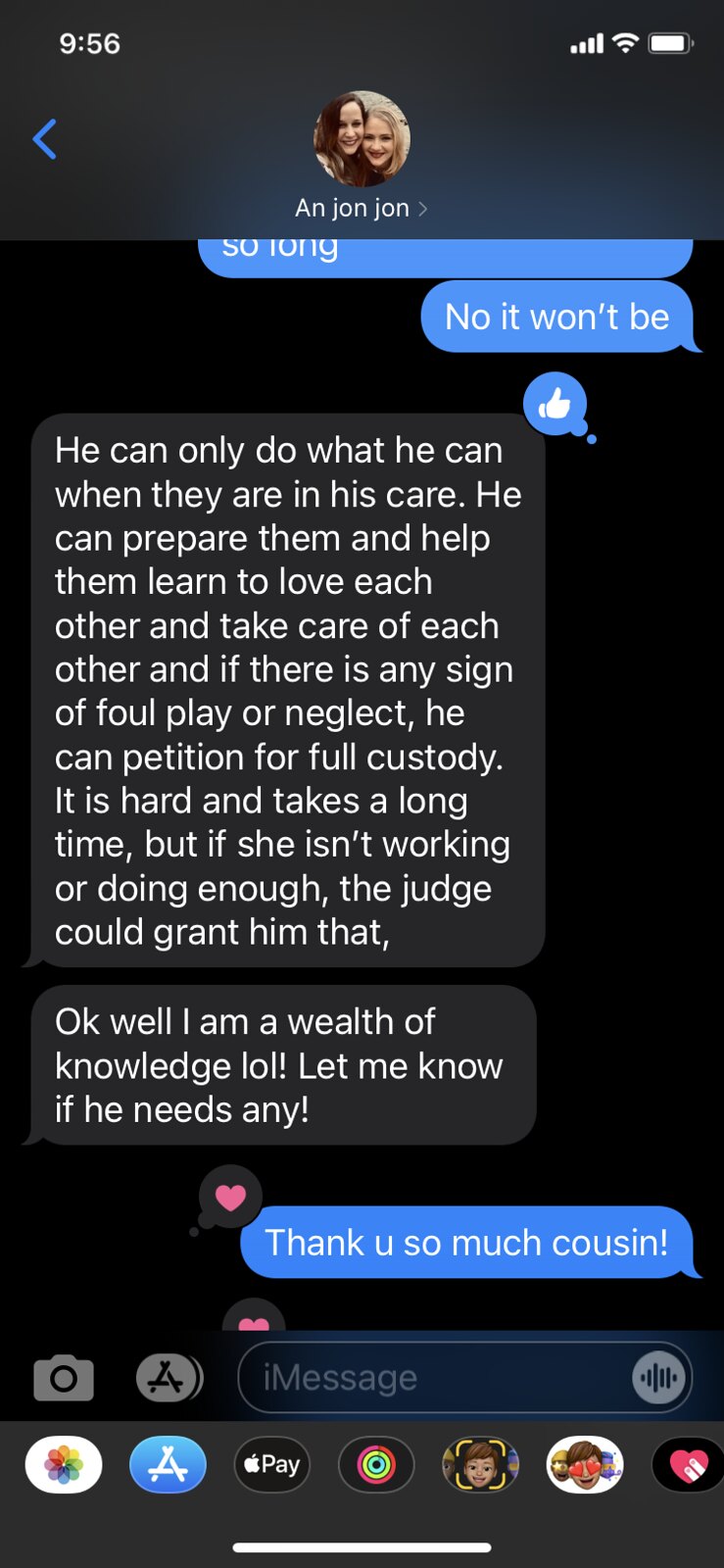The image is a screen capture from a phone displaying a text message conversation with a black background. At the top-center in white text, it reads "John John." On the top-left, a timestamp reads "9:56," and in the upper-right corner, connectivity bars, a Wi-Fi symbol, and a battery icon are visible. Just beneath, there’s a dark blue horizontal bar with a round photograph of two people and an unreadable name.

The conversation consists of light blue chat bubbles with white text and black chat bubbles with white text. The first visible message in a light blue bubble says, "so long, no it won't be." Following this, a lengthy message in a black bubble reads, "He can only do what he can when they are in his care. You can prepare them and help them learn to love and take care of each other. If there is any sign of foul play or neglect, he can petition for full custody. It is hard and takes a long time, but if she isn't working or doing enough, the judge will grant him that. Okay, well, I'm a wealth of knowledge, LOL. Let me know if he needs any." This text is followed by a red heart emoji.

In response, another light blue bubble says, "Thank you so much, cousin," which includes a heart emoji. Below this text bubble, there’s an icon of a camera, an icon of an 'A,' and an "iMessage" bar where the next message would be typed. The bottom edge of the black background shows a row of horizontal icons, and centered at the base is a horizontal white bar extending three-quarters of the screen's width.